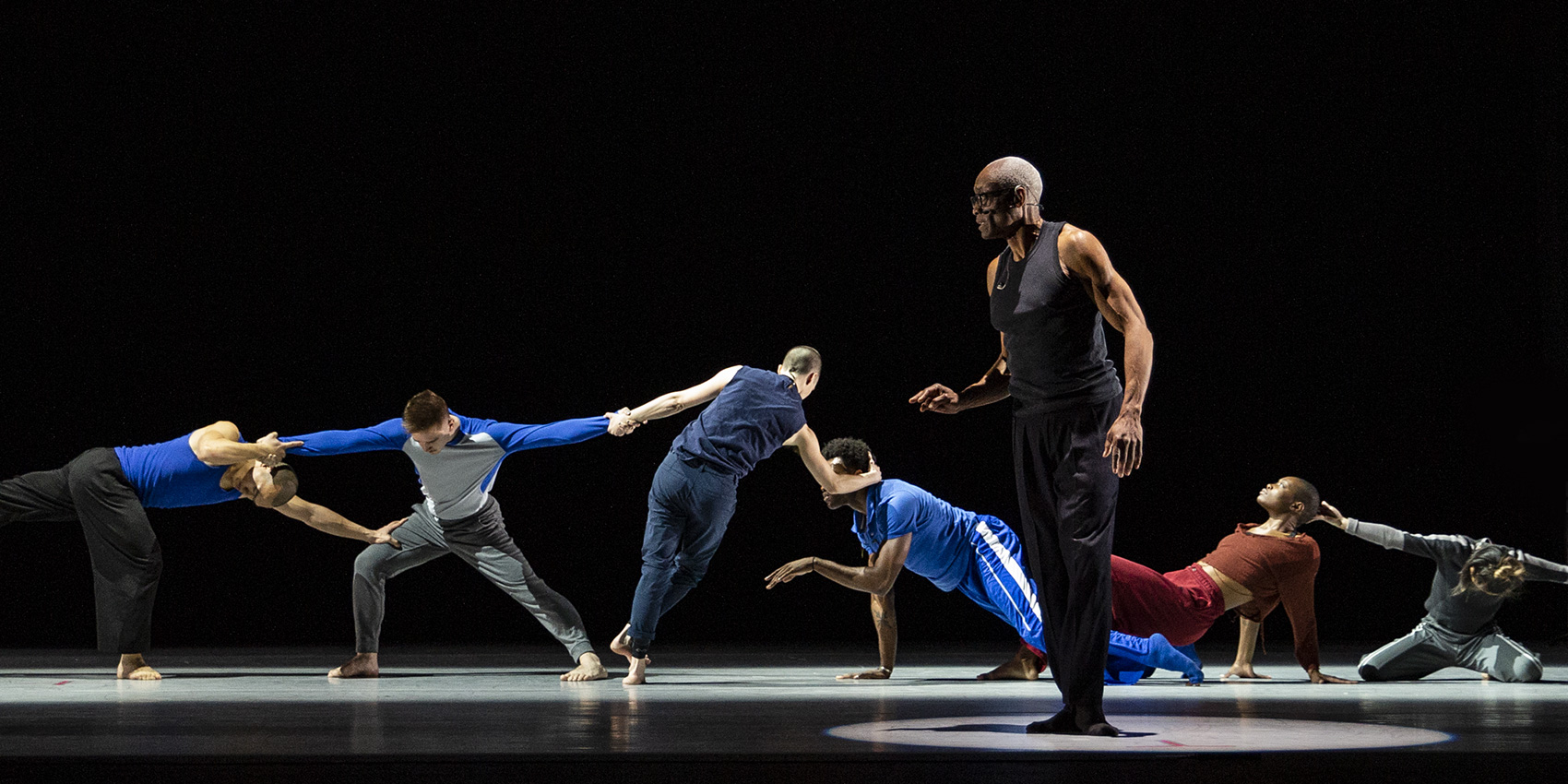This photograph, taken on a dimly lit stage, showcases a captivating dance performance featuring a diverse group of dancers illuminated by round spotlights. The background is a deep black, creating an intense contrast with the performers who are positioned centrally on the stage. The focal point is an older man of African descent, standing near the center of the stage. He is dressed in all black with a sleeveless vest and long pants, his short gray hair visible. His stance is powerful yet graceful; his right arm is bent at a 90-degree angle in front of him, while his left arm is slightly behind.

Surrounding him are six dancers interconnected in an intricate formation, each supporting and holding onto one another. To the left, a man in a blue tank top and black pants is balancing on his right leg, bent over at the waist. His outstretched arms grip the right arm of another dancer in a blue shirt, while his left hand secures this dancer's leg. This interconnected chain continues with the dancer in the blue shirt holding onto yet another performer clad in a blue tank top and blue pants. This individual has his back to the camera, standing on one foot and leaning to the right, his arm entwined around the head of another man of African descent who is on all fours.

Further back, another performer, a woman of African descent, is contorted on her feet and hands with her stomach facing upward. On the far right, a kneeling woman touches the back of her head, her head bent forward, and only the top visible from the camera's perspective. All the dancers are dressed in loose-fitting, flexible clothing such as tank tops, sweatpants, baggy pants, and cropped shirts, and they are all barefoot. The composition of the dancers, connected and supporting each other in various dynamic positions, creates a visually stunning depiction of unity and balance.